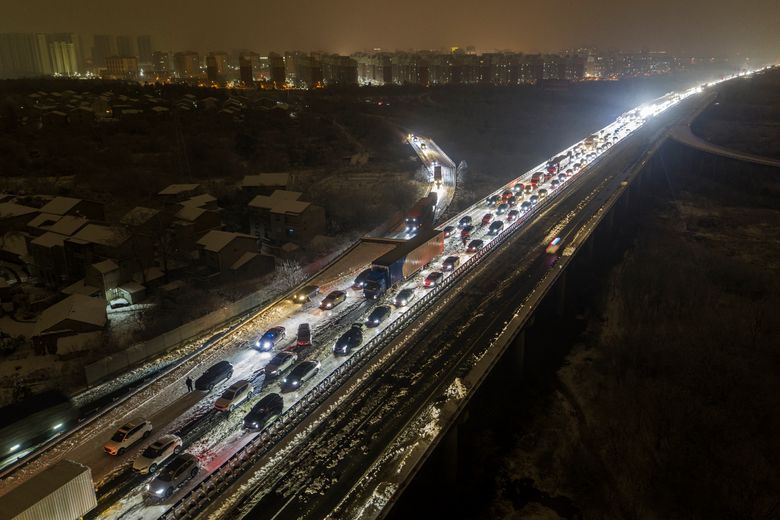The photograph captures a dreary night scene from a high vantage point, overlooking a snow-covered, congested highway. The highway, clearly a major route possibly an interstate, stretches diagonally from the bottom left to the top right of the image, with vehicles' headlights and taillights illuminating the otherwise dark and black foreground. The cars appear to be at a standstill, caught in a significant traffic jam, exacerbated by the unfavorable, snowy weather conditions. Flanking the highway, snow-draped rooftops and houses nestle in the dim light. In the hazy background, the cityscape with its skyscrapers and condominiums blurs into the foggy, brownish night sky, their lights barely piercing the gloom. The overall atmosphere is one of an arduous, cold commute under bleak, challenging conditions.